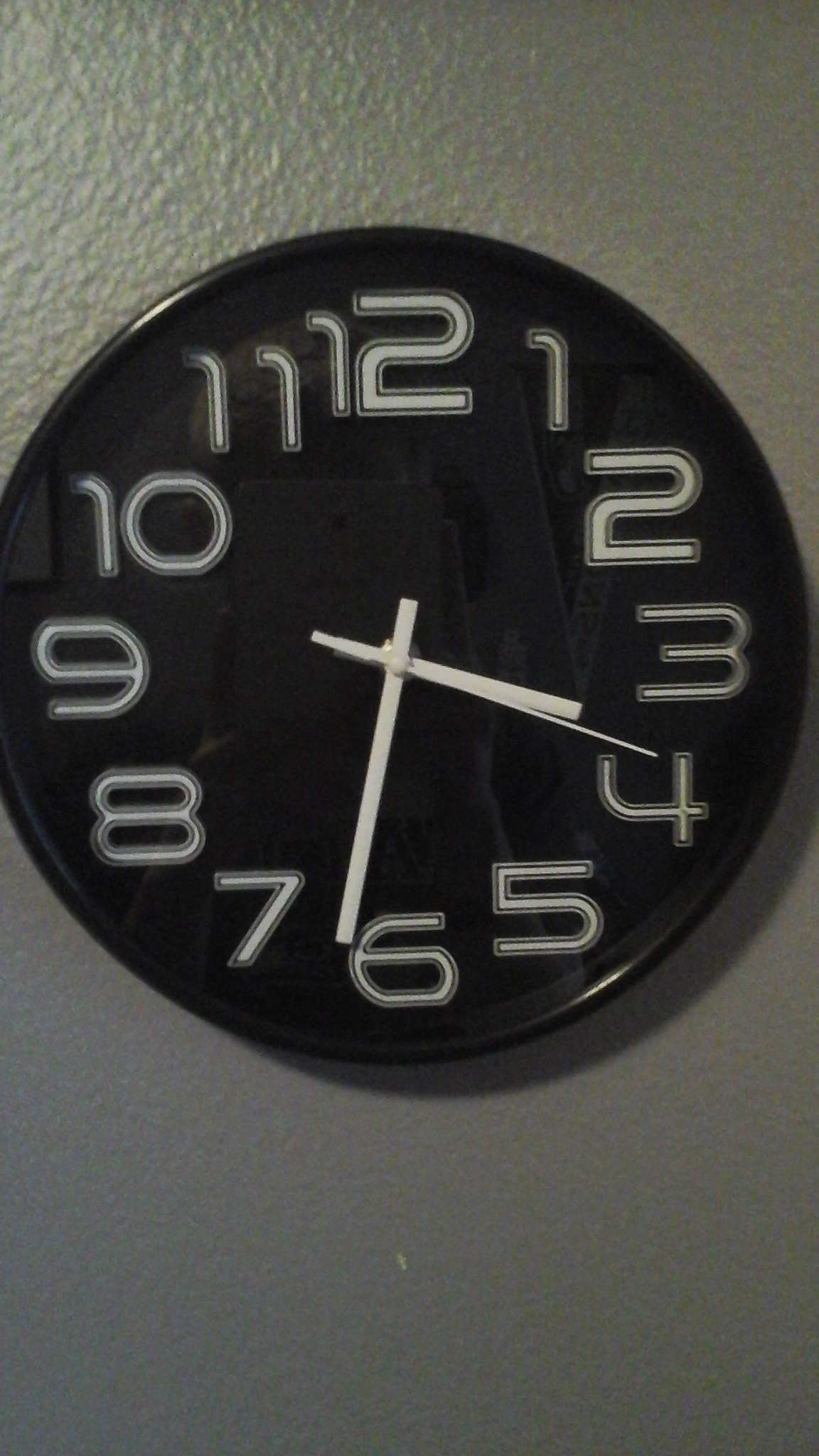This vertical image features a sleek, contemporary clock mounted on a textured gray stucco wall, exhibiting a pimpled finish. The disc-shaped clock is minimalistic yet striking, with a narrow black frame encasing a black face. Stylized white numerals, each outlined in a subtle gray hue, are prominently displayed against the dark background. The clock’s rectangular hour and minute hands, along with the pointed second hand, are also white, standing out conspicuously. The time is precisely set at 3:32. Positioned in the upper center of the frame, the clock is slightly cropped at the 9 o'clock position, adding an artistic touch to the composition.